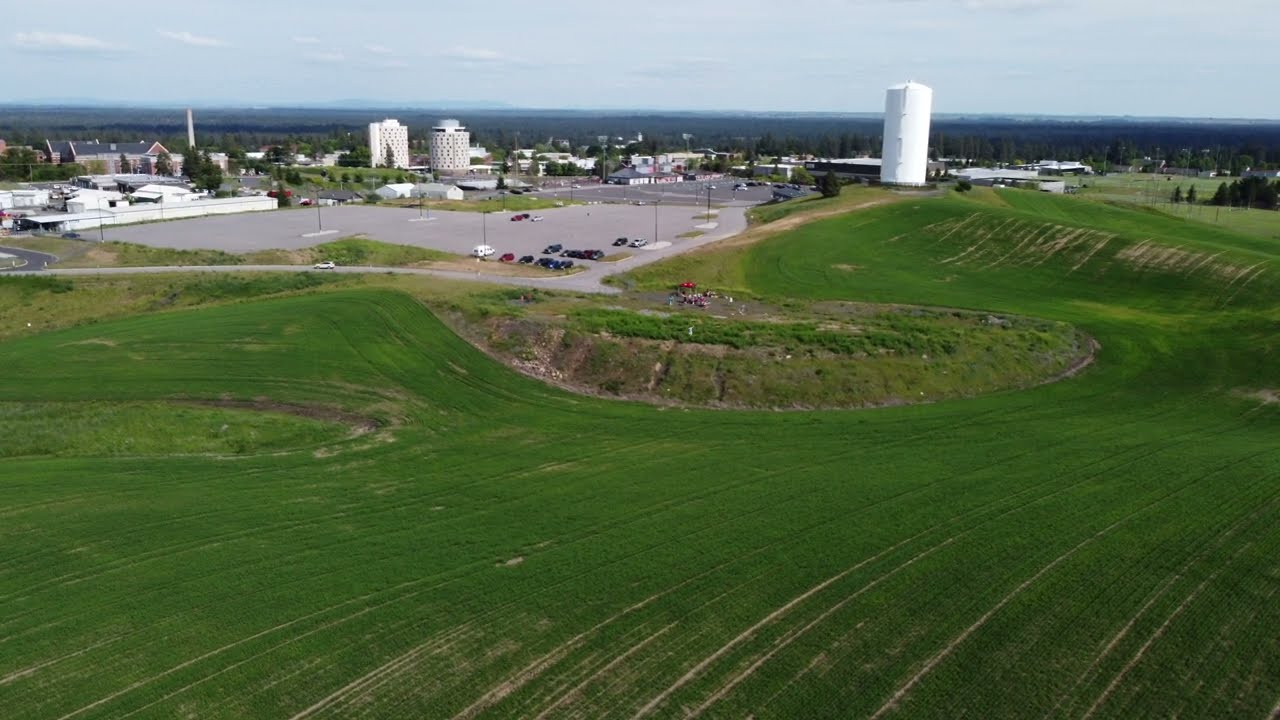In the image, we observe a vast, lush green field stretching across the foreground, characterized by well-manicured, short grass and gently rolling hills lined with uniform rows of dense foliage, indicative of farming activity. To the far edge of the field lies a large, gray concrete parking lot populated with several cars and flanked by various types of buildings, including a prominent white structure resembling either a grain elevator or water tower. Additionally, two rounded buildings stand in the central background of the parking area. Beyond these, the scene transitions into a sparse arrangement of buildings, possibly marking the outskirts of a small town or a rural area. In the upper left, a notable tall structure, potentially a church, is visible among the distant buildings, enhancing the rural town ambiance of the setting. A small group of people can be seen near the edge of the field, though their activity remains indeterminate. The serene composition of the field, parking lot, and distant structures is enveloped in a tranquil palette of green, white, blue, red, and gray hues.